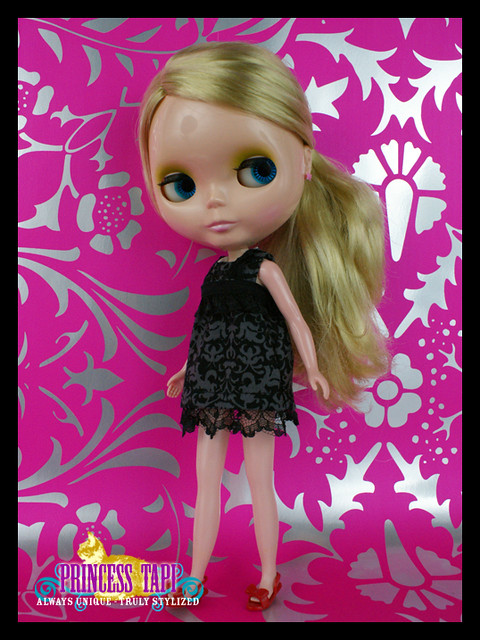The image depicts an advertisement for a doll named "Princess Tap," accompanied by the slogan "Always Unique, Truly Stylized." The doll features an exaggerated, elongated head with large, blinking blue eyes and a mature, adult-like face. She has voluminous, blonde hair styled in a ponytail that extends below her shoulders. Her outfit consists of a black lace nightgown paired with red heels adorned with ribbons. The doll stands against a decorative background with a silver and purple floral pattern, reminiscent of wrapping paper. At the bottom left corner of the image, there is a gold cat logo with the text "Princess Tap" displayed prominently, and underneath it, the tagline "Always Unique, Truly Stylized" is inscribed in smaller white font. The entire image is framed with a black border, completing the advertisement's polished look.